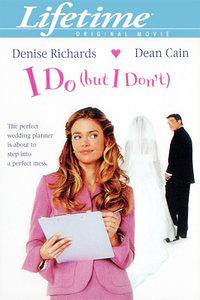The advertisement is a vertical rectangular image primarily set against a white background, with the top border colored blue. Within the blue border, large white letters spell out "Lifetime," followed by "Original Movie" in smaller letters beneath. Directly below this, on the white background, the names "Denise Richards" and "Dean Cain" are prominently displayed. 

The main focus of the image is a large picture of Denise Richards, standing and facing forward but with her eyes cast to the right. She has long, curly, brown hair and is dressed in a pink suit, holding a clipboard in her right hand and a pencil in her left. To her left, there are five lines of black text, difficult to decipher but possibly containing key information about the movie. To her right, there's an image of Dean Cain in a tuxedo, standing close to a bride in a wedding gown. Both are facing away, with Dean Cain glancing back towards Denise Richards. 

In large pink letters, the movie title "I Do, But I Don't" appears prominently, hinting at romantic and possibly comedic elements. Additional text near the bottom indicates the tagline: "The Perfect Wedding Planner is about to make a perfect mess." The overall composition makes for an intriguing and detailed promotion of the Lifetime Original Movie featuring Denise Richards and Dean Cain.